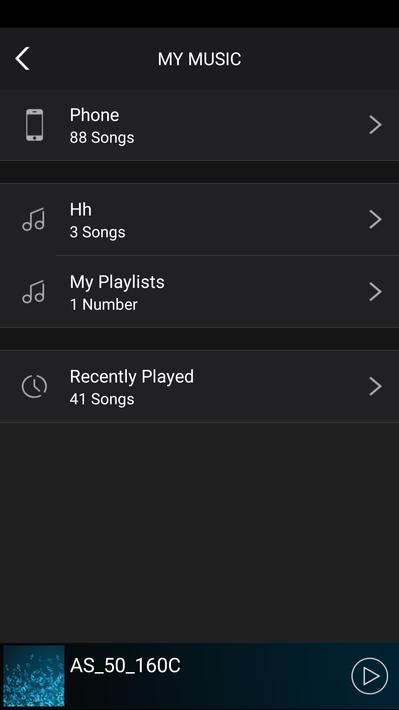Screenshot of a digital music library interface displayed on a black screen. At the top, there's a back arrow icon followed by the text "My Music." Below it, there's an image of a phone labeled "Phone" with "88 songs" next to it. To the right, there's an arrow icon next to the text "H" (lowercase "h"), and "3 songs" alongside another arrow icon with a music note. The section "My Playlist" appears with "1" beside it and an arrow icon, followed by a clock icon with the text "Recently Played 41 songs". At the bottom left corner, there's a blue square icon with blue bubbles on it and the text "AS_50_160C". Adjacent to it is a play button set against a dark grayish-blue background.